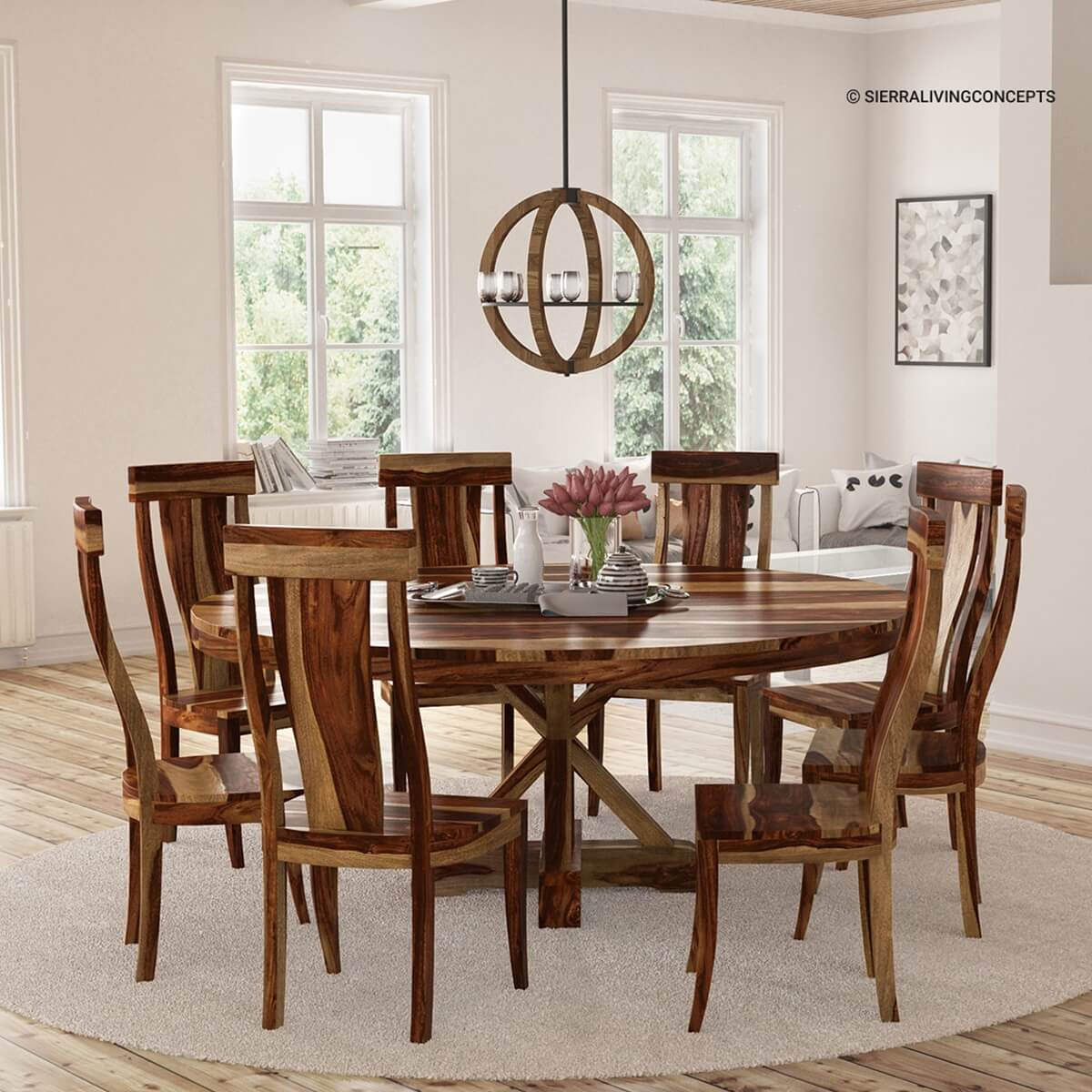This image captures a dining room with a striking wooden table that showcases a handcrafted, two-toned design of dark mahogany and light oak wood, surrounded by eight matching wooden chairs. The table is adorned with a clear vase holding vibrant pink flowers and a tray featuring a teapot, creamer, sugar, and a small coffee mug. Additionally, there's a white vase completing the tabletop arrangement.

Above the dining table, a modern chandelier hangs, designed as a cylindrical wooden structure with eight candle-like light bulbs. The dining set rests on a round beige rug atop what appears to be an unfinished oak floor. 

In the background, the room opens up to reveal a cozy area with a couch adorned with a white pillow featuring black splotches and a few books placed on the windowsill. There are two large windows without curtains, offering a beautiful view of lush green trees outside. A gray and white abstract painting, with the words “Sierra Living Concepts” inscribed at the top right, adds a modern touch to the white wall.